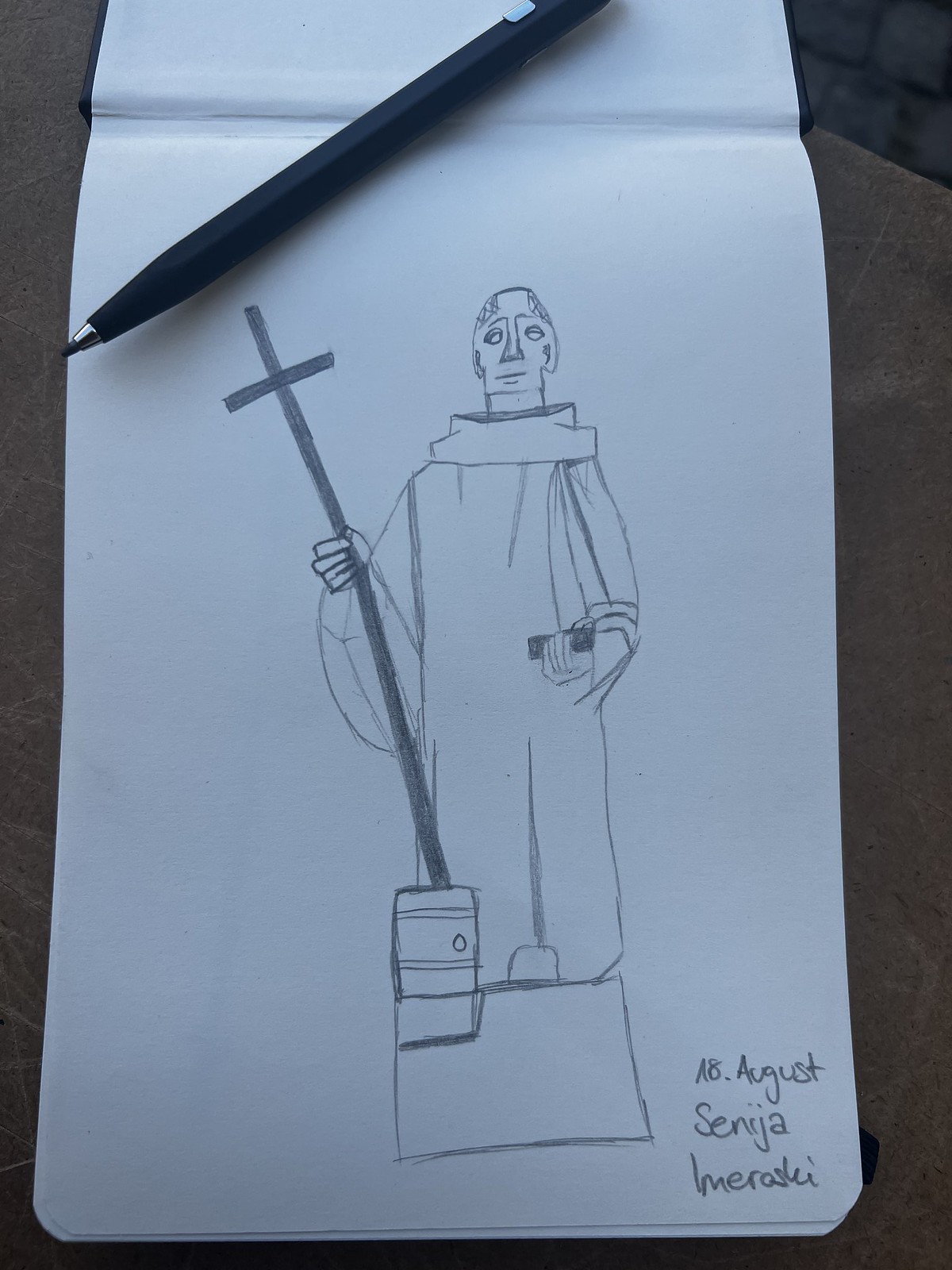This photograph captures a detailed drawing in an open white sketchbook. The upper portion of the image clearly shows several pages bound together, characteristic of a sketchbook. The artwork within the sketchbook depicts a religious figure, possibly a saint or a Catholic monk. The figure is dressed in traditional monk robes and has a distinct tonsure hairstyle—bald on top with a ring of hair around the head.

In the figure's left hand, they hold a long black cross, symbolizing their religious devotion. In the right hand, there is a rectangular, gray object, likely a book or another significant item. At the bottom of the sketch, the artist has signed and dated their work: "Señiaimeraski," dated August 8th.

Additionally, the black pencil used to create this piece is visible at the top of the photograph, easily identifiable by its metal ferrule and the exposed pencil lead. The meticulous detail in the drawing and the thoughtful inclusion of the artist's tools add depth to this captivating image.